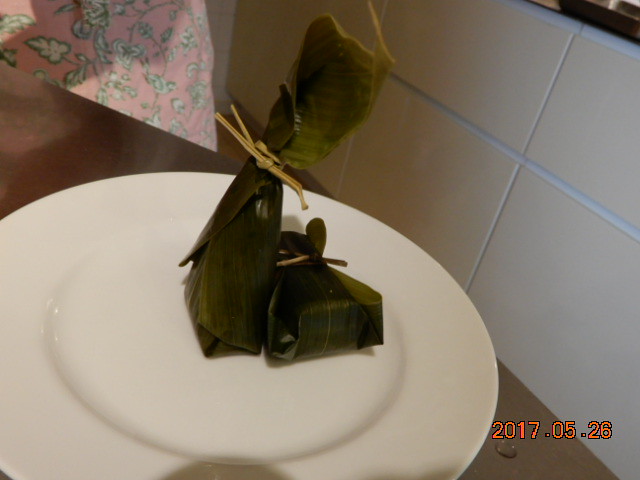The image features a round white plate set on a brown table, displaying two uniquely wrapped food items, presumably encased in banana leaves. The food parcels have a long, triangular shape, one standing upright and the other laid flat, each secured with a tan cord. In the background, white kitchen panels and grout suggest a modern kitchen setting. To the upper left of the plate, there is a pink item with a floral leaf pattern, possibly a piece of fabric or paper. This photograph, dated May 26, 2017, captures a detailed and textured culinary presentation.